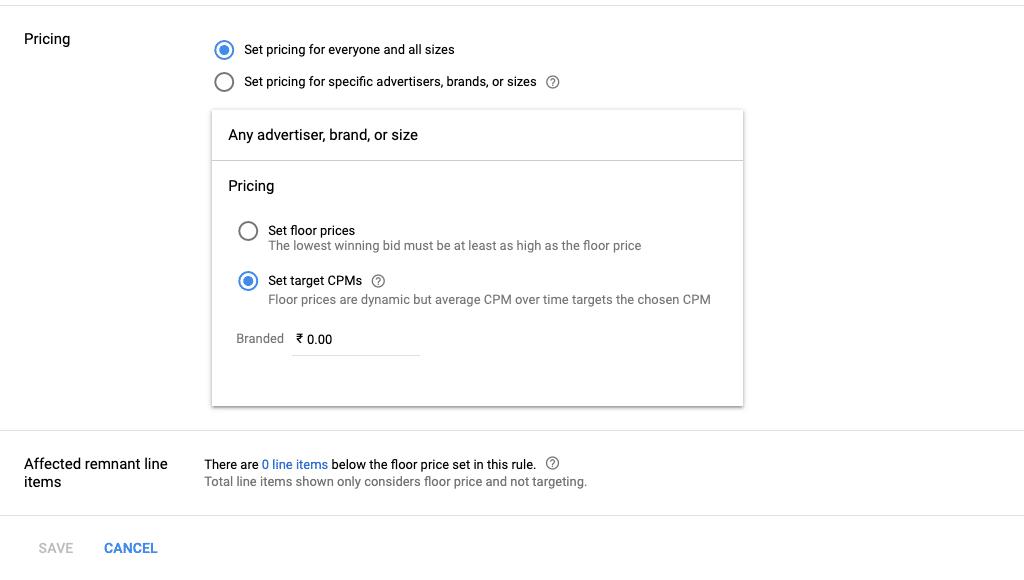**Detailed Description for a Website Pricing Configuration Interface**

This is a horizontal website interface, positioned on the far left-hand side, specifically designed for setting pricing options. The interface header is labeled "Pricing."

Below the header, there are two primary options:

1. **Set Pricing for Everyone in All Sizes** 
2. **Set Pricing for Specific Advertisers, Brands, or Sizes**

Underneath these options is a prominent box.

**Box Header**: "Any Advertiser, Brand, or Size Pricing"

**Box Content**:
- **Set Floor Prices**: It specifies that the lowest winning bid must be at least as high as the floor price.
- **Set Target CPMs**: It explains that floor prices are dynamic but the average CPM over time targets the chosen CPM.

Next to "Branded" is a currency symbol, which is challenging to identify, followed by "0."

At the bottom of this box, it says, "Affected Remnant Line Items. There are zero items below the floor price set to this rule. Total items shown only consider the floor price and not targeting."

In the bottom left-hand corner of the interface, there are two buttons:
- The "Save" button, which is gray and reads "SAVE" in all capital letters.
- The "Cancel" button, which is blue and reads "CANCEL" in all capital letters.

This configuration interface is likely used by someone responsible for pricing or budgeting within a company, providing a detailed view and control over pricing settings on a website.